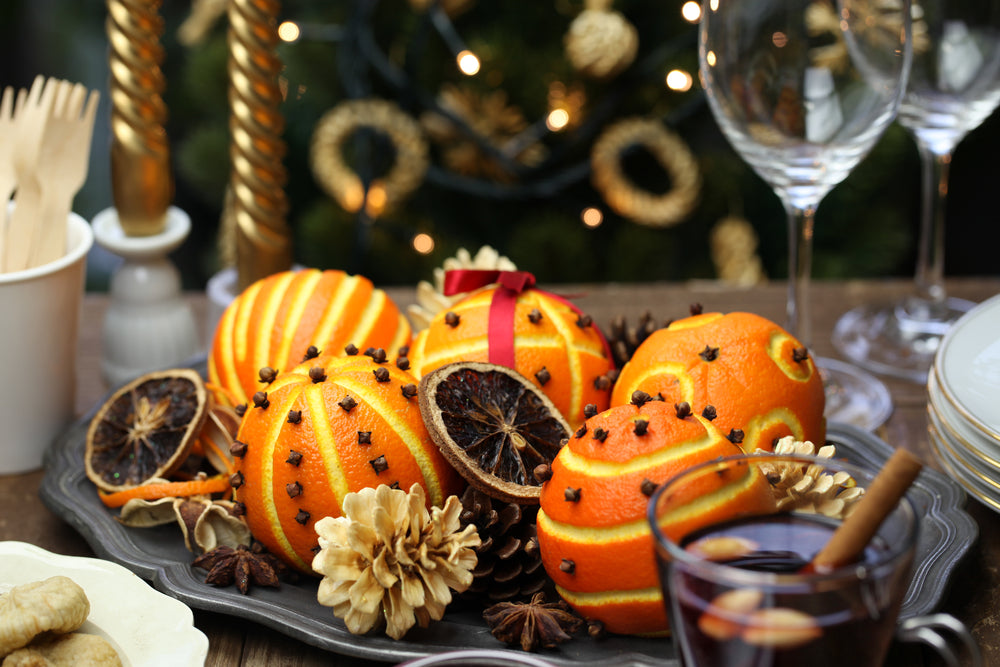The image is a detailed color photograph capturing a festive tabletop scene. Central to the composition is a dark gray or black oval platter adorned with intricately peeled oranges, each decorated with cloves, creating a potpourri effect. Nestled among the vibrant oranges are both white and brown pine cones, as well as slices of dried blood orange. Surrounding the platter are various glassware, including two empty wine glasses and a glass cup containing mulled wine with a cinnamon stick. There are also ceramic white candle holders featuring gold spiral tapered candles, contributing to the warm, celebratory ambiance. A stack of plates with gold rims is positioned to the right, complementing the overall aesthetic. In the background, a glimpse of a Christmas tree hints at a holiday setting. The table itself is wooden, creating a rustic contrast to the elegant tableware and festive decorations. The colors in the image range from orange and gold to black, off-white, light brown, and yellow, enhancing the detailed, cozy atmosphere of the scene.